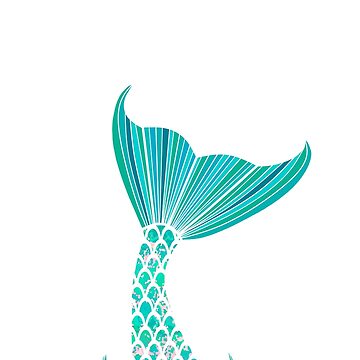This small, flat illustration features a vividly colored mermaid tail, rendered with stylized scales in shades of green, teal, and blue, set against a stark white background. Positioned vertically and curving slightly from left to right, the tail emerges from the lower part of the image, with its expansive fin dominating the scene. The meticulously detailed scales and striped band's gradient hues evoke an aquatic theme, making the tail appear almost lifelike in its simplicity. The tips of the lateral fins, barely visible, hint at the rest of the creature’s form, further emphasizing the intricate beauty of this 2D drawing that is both minimalistic and bright.